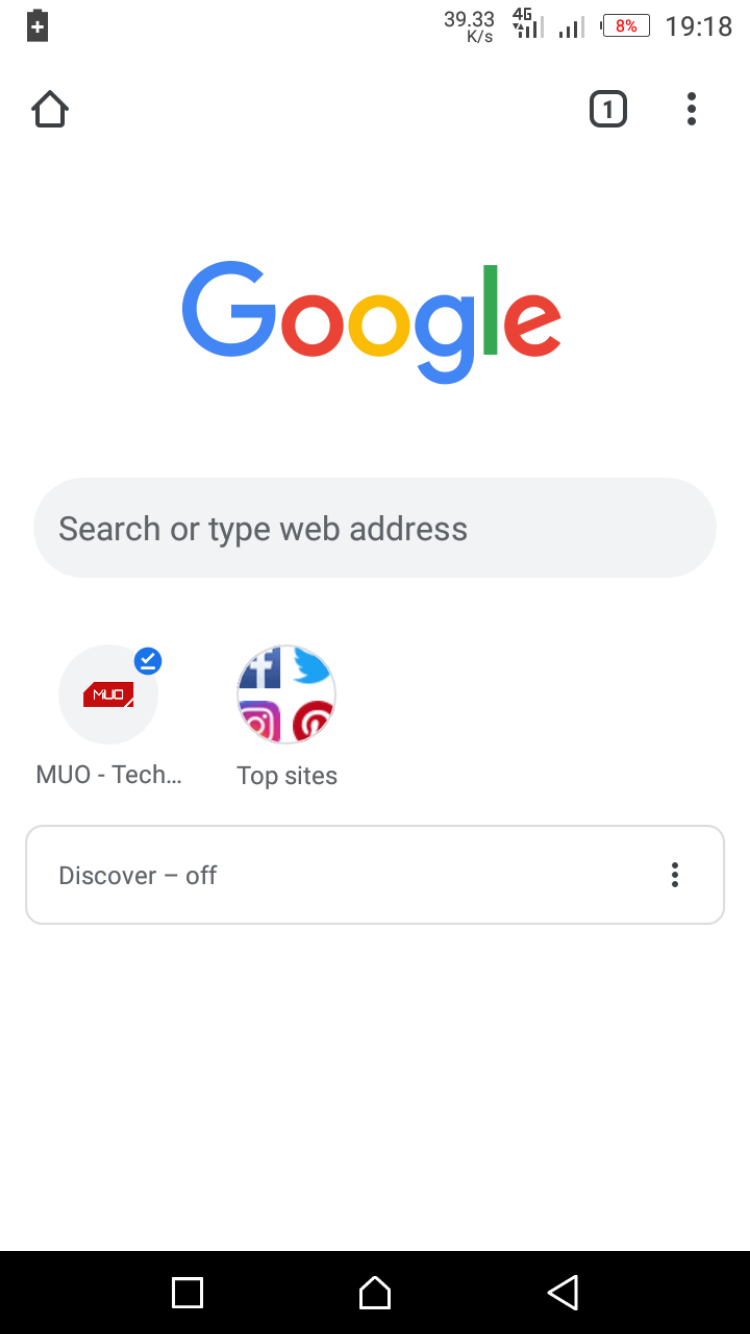This detailed description depicts an iPhone screen. The battery indicator is at a critically low 8%, displayed in red. The time shown is 19:18, and the device is connected to a 4G network. To the right of the screen is a home button, while to the left appears to be a battery icon with a plus sign.

Directly beneath the 8% battery indicator is a notification marked by the number one, highlighted with a blue outline and accompanied by three blue dots. This is outlined in black with three corresponding black dots.

Dominating the center of the screen is a large Google logo, characterized by its colorful letters (a blue G, red O, gold O, blue G, green L, and a red E). Below the logo lies a substantial gray search bar with rounded edges, prompting users to "search or type web address."

Further down, the text "MUO tech" is displayed. Adjacent is a red circle containing an image, and above it, a smaller blue circle with a checkmark. Next to this, the label "top sites" inicates frequently visited websites, represented by iconic logos: a recognizable "F" for Facebook, the bottom portion of the Twitter bird, a fragment of the Instagram logo, and a part of the red Pinterest circle.

Below these icons is a solid white bar displaying the message "discover is off." Additionally, three dots are visible. At the very bottom of the screen, a black bar contains three unspecified icons.